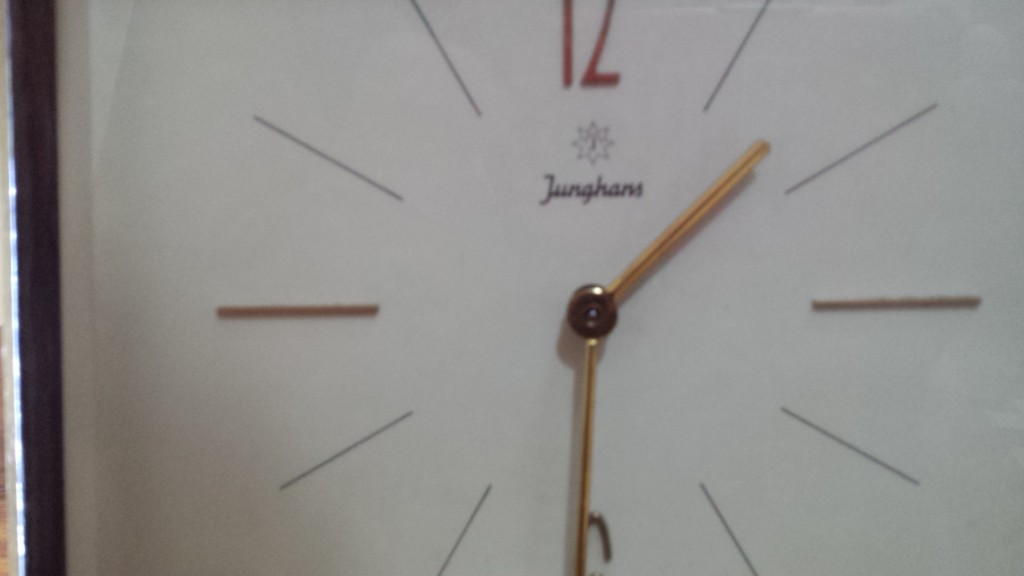This is a highly detailed, up-close photograph of a square-shaped clock with a white face. The clock features simple gold-colored bar-style minute and hour hands, both positioned around the 1:30 mark. The clock face is adorned with a notable red "12" at the top and a partially visible "6" at the bottom. There are red lines marking the 3 and 9 o'clock positions, while thinner black lines indicate all other hours. Beneath the red "12" is the brand name "JUNGHANS" written in cursive script, accompanied by a small star logo with a 'J' in the center. The image captures a reflection of light in the far left corner, shining off the clock's raised black frame.